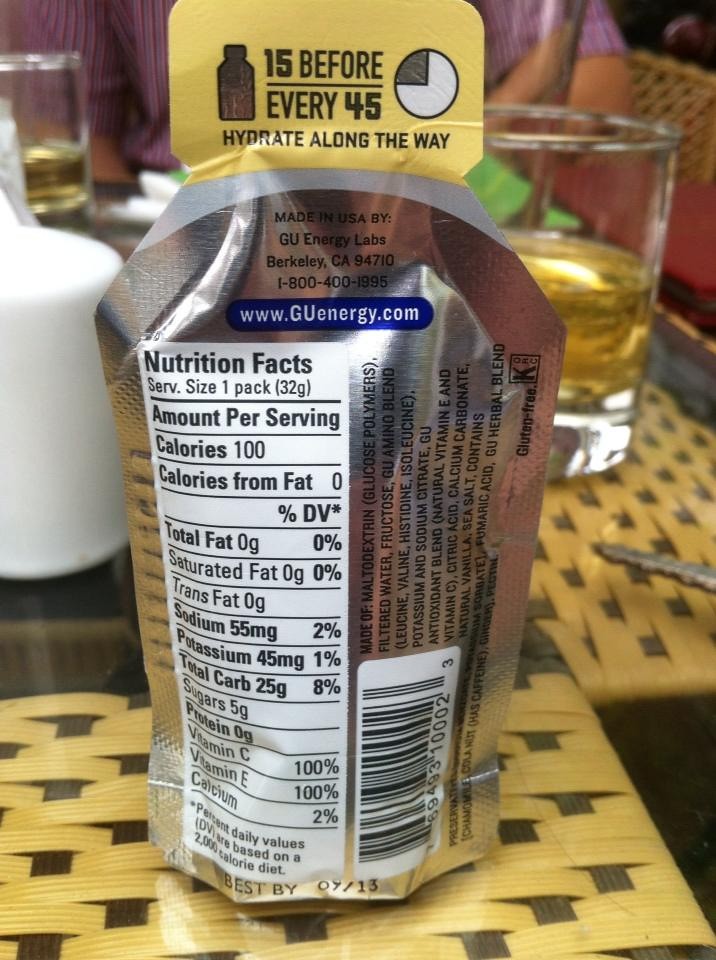This image depicts the back of a silver, rectangular pouch resembling a Capri Sun, likely containing an energy drink. The pouch stands on a gold and gray woven placemat, possibly outdoors, and has a yellow tab at the top with a silhouette of a bottle and the text "15 before every 45 - hydrate along the way" written horizontally. The top of the pouch features a blue rectangular banner displaying the website www.guenergy.com. On the left side of the pouch is a white vertical nutrition facts box listing 100 calories, 55mg of sodium, 45mg of potassium, and 25g of total carbs, with only 5g of sugars, flanked by a list of ingredients written vertically and a UPC code. Text at the bottom indicates it's made in the USA by DU Energy Labs in Berkeley, California, with a contact phone number and additional website duenergy.com. Adjacent to the package in the background, there's a glass containing a liquid and a white container, suggesting this is a beverage intended for hydration during physical activities.